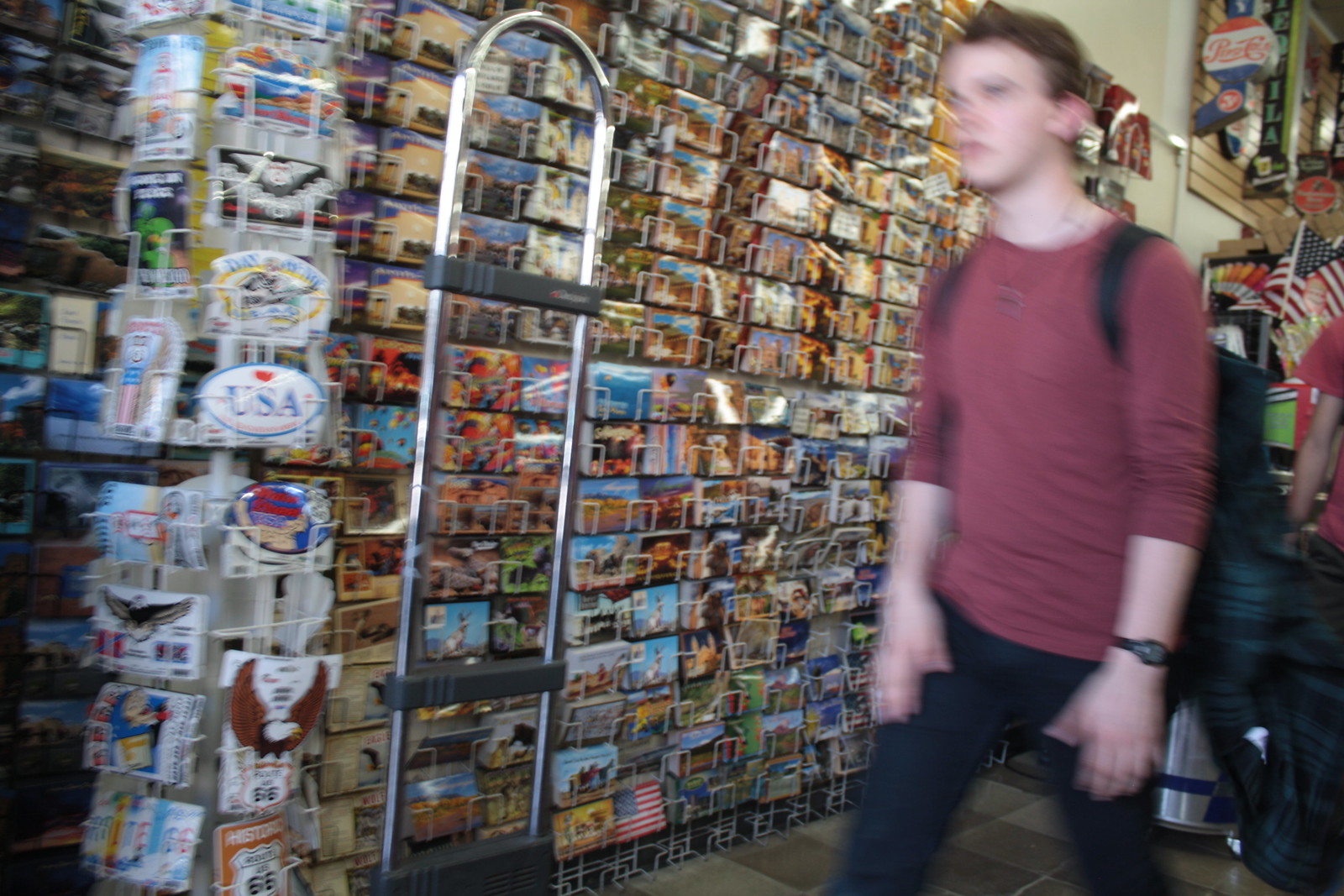This photograph captures a young Caucasian man walking through a store, slightly blurred, suggesting he is in motion. The image is about 20-30% wider than it is taller. The man has short brown hair and a somber expression, wearing a maroon long-sleeved shirt rolled up to his forearms, dark blue jeans, and a black wristwatch on his left hand. He is also carrying a black backpack. He appears to be walking past a large postcard display situated on the left side of the image, which features a diverse collection of postcards in various shapes and colors, including designs with American flags, wings, and scenic locales. Adjacent to the postcard display is a rack with stickers, one of which reads “Heart USA.” To the right side of the image, a dolly and a metal implement can be seen, hinting at store merchandise activities, while in the background, a section of an American flag and another store patron in a red t-shirt are partially visible. A security bar is also present, suggesting theft prevention measures.